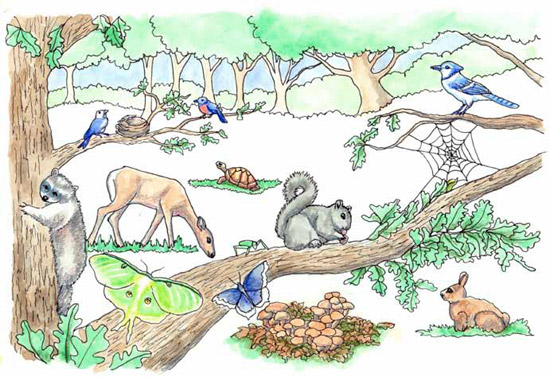The image depicts a vibrant, cartoon-style forest scene reminiscent of a children's coloring book. The artwork, likely created with colored pencils or crayons, features a variety of forest animals and insects, all meticulously colored within the lines. 

On the left, a gray raccoon climbs a tree, with two bluebirds perched near a nest on its branches. Below them, a majestic deer stands gracefully. In the center of the image, a turtle sits on a grassy patch, while two butterflies flutter nearby—one predominantly green and yellow with brown dots, and the other blue with gray accents. A gray squirrel is perched on a branch above a cluster of mushrooms at the ground level.

To the right, a vivid blue jay is visible in the upper corner on a branch. Nearby, a spider web stretches between tree branches with a green bug nearby. At the bottom right, a brown rabbit sits quietly. The background is filled with lush green trees, creating a dense forest backdrop, while the sky appears a clear blue. This charming illustration captures the essence of a lively woodland scene, blending detailed line art with warm, colorful hues.